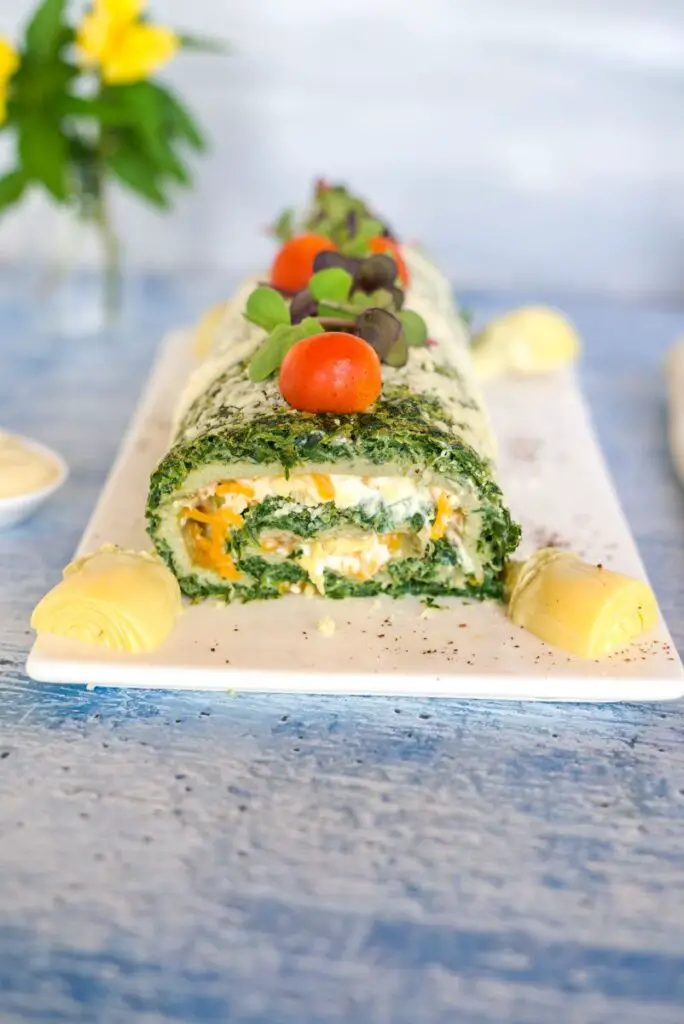In this vibrant foodie photograph, a carefully arranged appetizer is laid out on a rectangular, white cutting board that rests upon a table in shades of blue, light pink, and cream, likely made of wood. The main focus is a meticulously layered wrap, resembling a log roll of cheese stuffed with various ingredients. The wrap is cut to reveal its enticing filling, which includes layers of white cheese, orange cheddar cheese, and finely shredded spinach or another green vegetable. Adorning the top of the wrap are an array of fresh garnishes: small cherry tomatoes, sprigs of herbs, and maybe small pieces of artichoke heart or another light yellow vegetable. The garnishing extends along the center of the wrap, while the background transitions to a soft blur, giving it an artistic touch. In the backdrop, a glass vase holds two charming yellow flowers with muted green leaves, enhancing the overall elegance of the setting, indicative of a refined appetizer presentation for a stylish event.